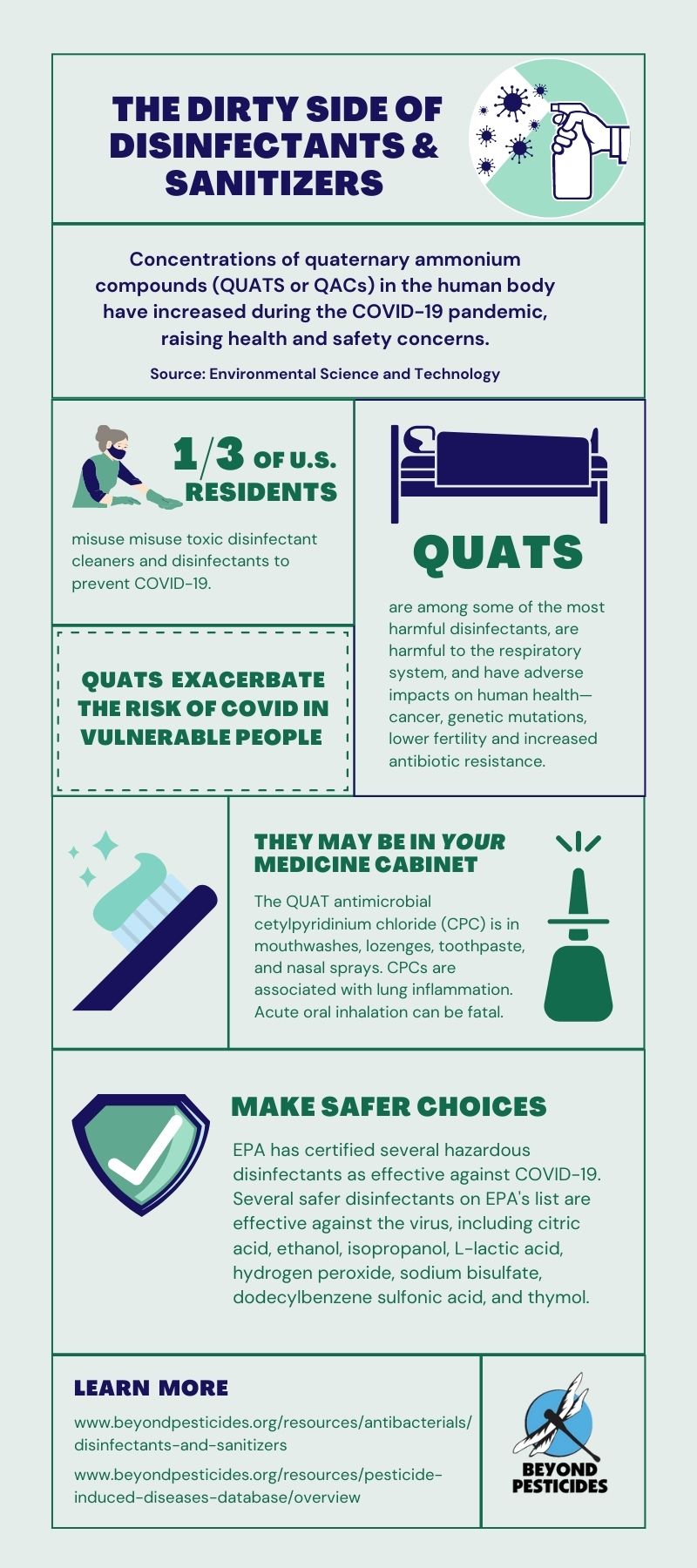The poster titled "The Dirty Side of Disinfectants and Sanitizers" features a detailed infographic. On the right side, a graphical image depicts a hand holding a white spray bottle, releasing virus particles represented as ball-shaped entities with many tails sticking out. Below the title, the poster highlights a significant concern: the concentration of Quaternary Ammonium Compounds (QUATs or QACs) in the human body has increased during the COVID-19 pandemic, raising serious health and safety concerns. A woman wearing a blue mask is depicted near the bottom, where it reveals that one-third of U.S. residents misused toxic disinfectant cleaners in an attempt to prevent COVID-19. The poster further explains the health risks associated with QUATs, which include respiratory problems, cancer, genetic mutations, lower fertility, and increased antibiotic resistance. These compounds are commonly found in household items such as mouthwashes, lozenges, toothpaste, and nasal sprays, posing additional health risks like lung inflammation and acute oral inflammation. The poster encourages making safer choices and notes that the EPA has certified several hazardous disinfectants that are effective. For more information, the poster directs viewers to a website and features a logo for Beyond Pesticides with a dragonfly in a blue circle.